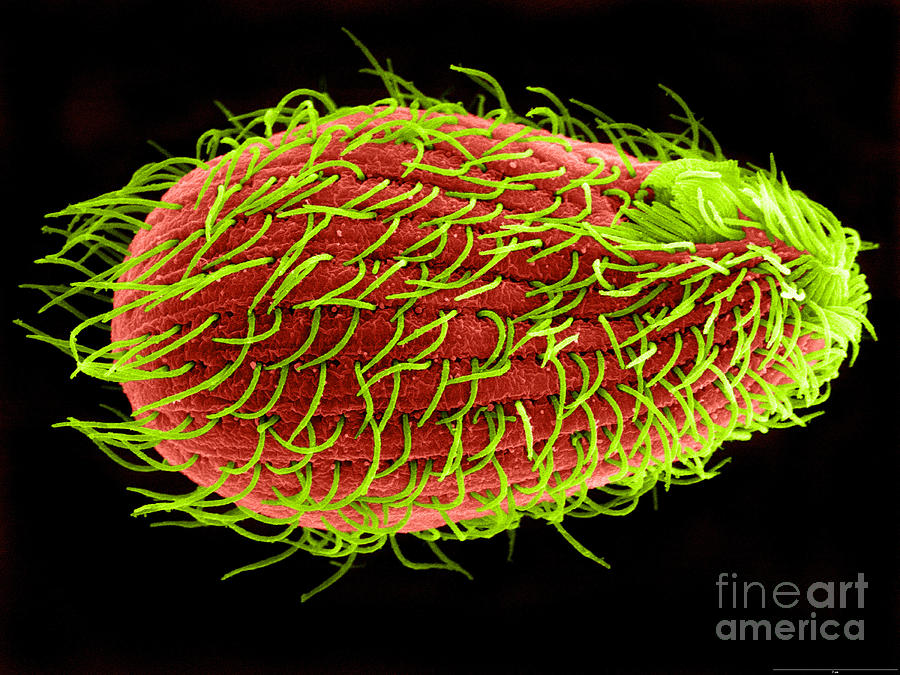This digital artwork, identified by the "Fine Art America" watermark in white on the bottom right corner, features a surreal, highly detailed image of a red, seed-like structure against a stark black background. The centerpiece of the image, which takes up the majority of the canvas, resembles an electron micrograph of a seed that has been post-processed into color. The seed, colored in deep red and maroon hues, has prominent channels running along its length. Emerging from the surface are clusters of bright, lime-green tentacle-like hairs that are sparsely distributed across most of the seed but form denser clusters near the narrow end, creating an effect reminiscent of a mohawk. The vibrant, almost neon green hairs and the rich red of the seed contrast strikingly with the solid black background, emphasizing the alien and intricate nature of the subject.